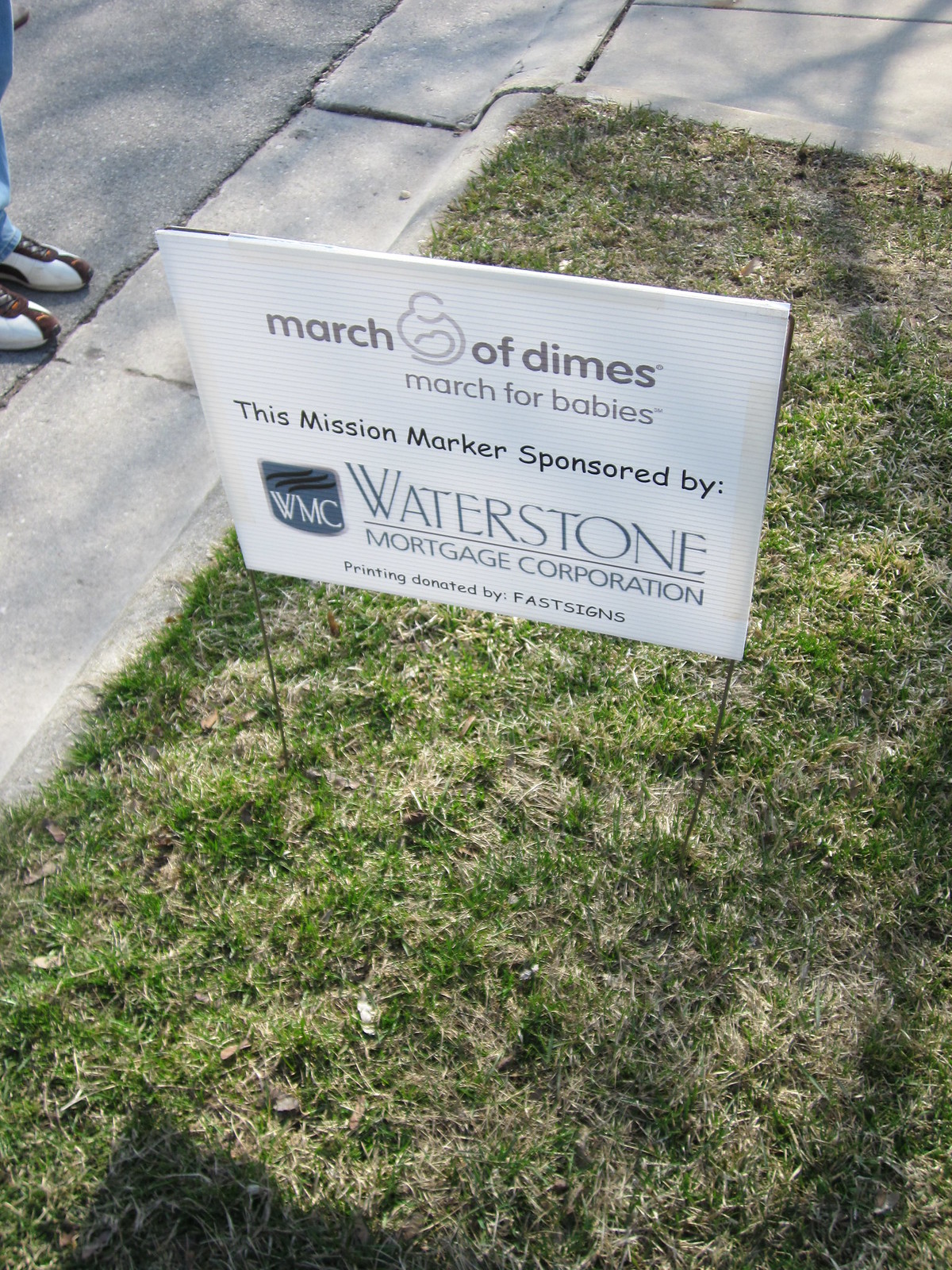This photograph captures an outdoor scene featuring a white yard sign staked into a grassy area near a walkway or street edge. The top part of the sign prominently displays the words "March of Dimes, March for Babies" in gray, accompanied by the organization’s logo—a circular emblem depicting a mother holding a baby. Below this, the message reads, "This mission marker sponsored by Waterstone Mortgage Corporation," with the logo for Waterstone Mortgage displayed as a blue shield featuring white letters "WMC" and three black lines at the top. Additionally, it notes, "Printing donated by Fast Signs." Off to the top left corner of the image, there's a partial view of a person’s jeans and shoes, with the shoes being white with brown accents, possibly Pumas. The background includes a glimpse of pavement and possibly a driveway at the edge of someone's lawn.